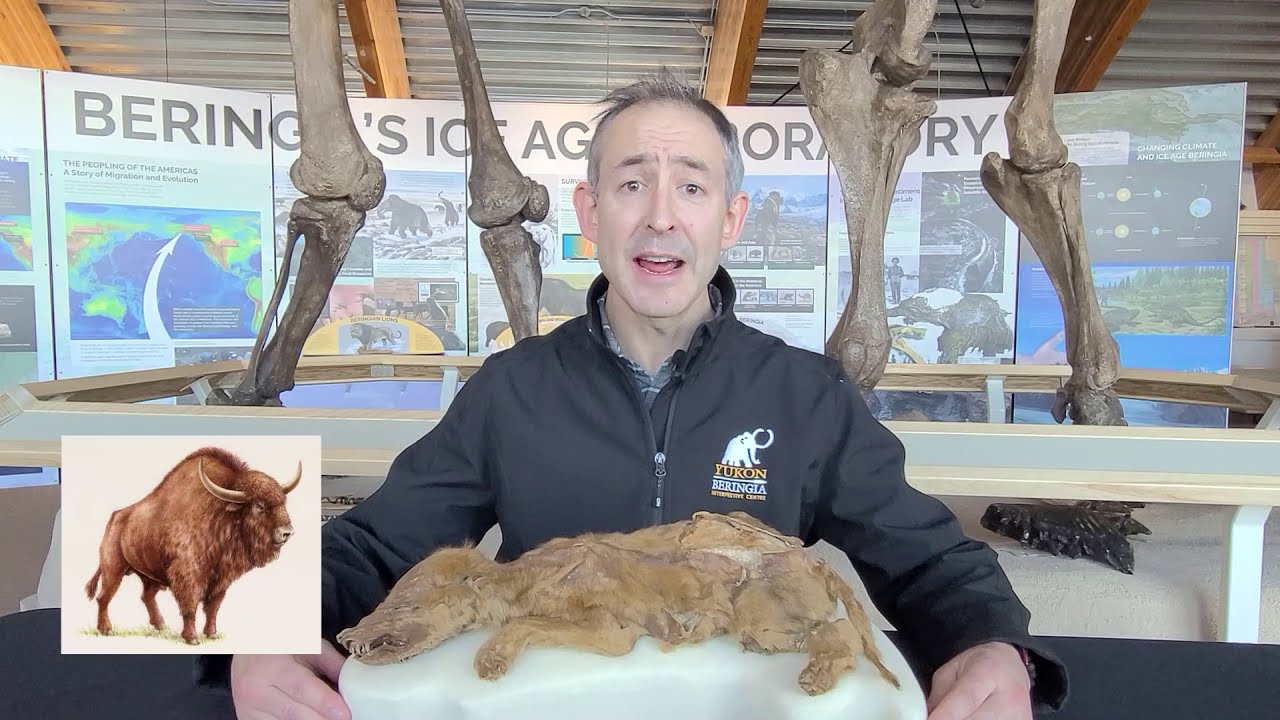In this landscape photograph, a Caucasian man with gray hair, dressed in a black zip-up hoodie adorned with a white and yellow logo that reads "Yukon Beringia," is engaging with the camera while presumably explaining a museum exhibit. He stands in front of a white sheet that showcases the preserved carcass of a woolly mammoth, with the remains arranged prominently in front of him. To the lower left corner of the image, there is a detailed sketch of a woolly mammoth, while behind him, various skeletal remains and colorful signage, featuring blues, reds, greens, and yellows, provide educational context about the Ice Age. The signage is sectioned into multiple vertical panels, depicting images of animals, weather patterns, and additional informative text.